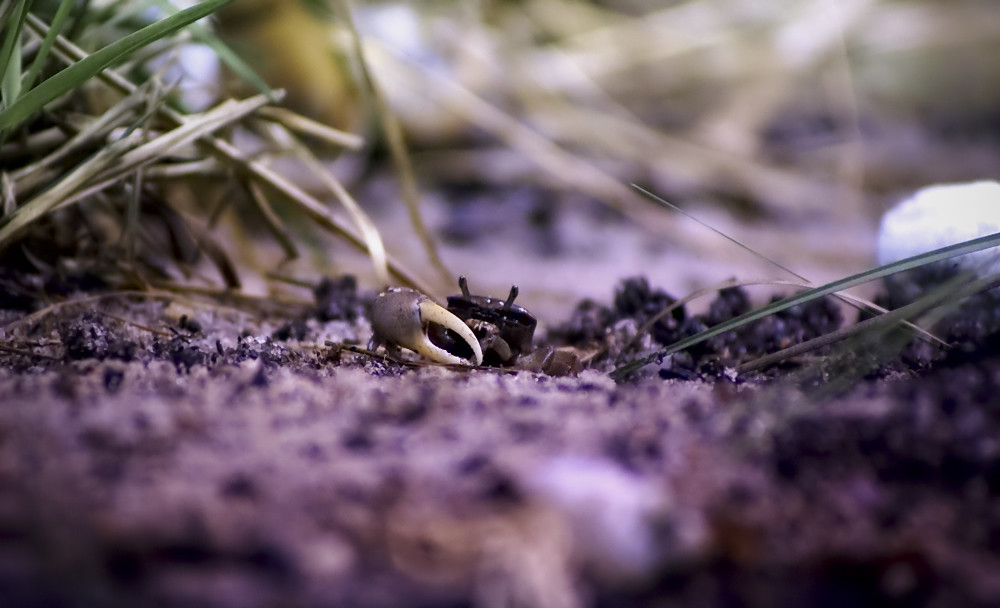This image is a macro photograph captured at ground level, featuring a detailed scene of black and tan dirt with scattered elements of nature. The focal point of the image is a tiny crab situated in the very center, its shell dark-colored with a noticeable lighter gray claw that has beige cream-colored snappers. The claw and the crab’s body stand out against a backdrop that is largely out of focus, creating a blurred ambiance suggesting a garden or wooded area. To the left of the crab, several greener and withered blades of grass rise from the dirt, while on the right, a green palm-like leaf extends from the edge of the frame. In addition to this, a small, rectangular brown object with antennas can be seen near the claw, hinting at another insect. The photograph, taken during the daytime, captures a small, vibrant ecosystem with fine details in the center fading into a softly blurred, natural background.